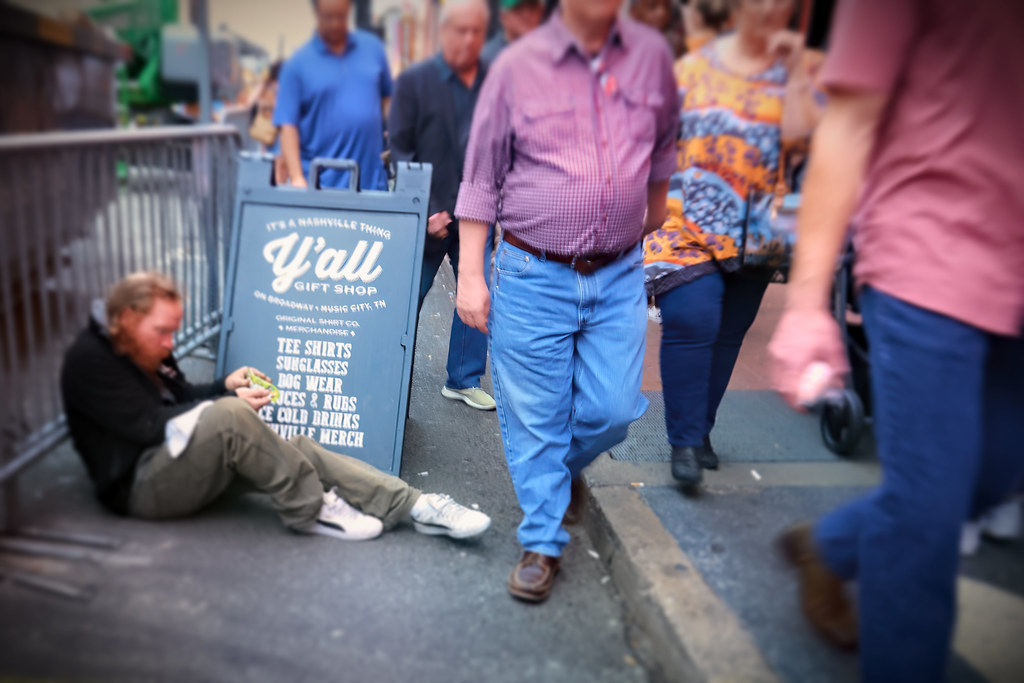The image captures a bustling street scene. On the far left of the frame, there's a metal barricade with a blue and white sign leaning against it, advertising a Nashville-themed gift shop offering t-shirts, sunglasses, dog wear, juices and rubs, ice-cold drinks, and other merchandise. A man with a long red beard and hair, dressed in a black jacket, khaki pants, and white sneakers, is sitting on the ground against the barricade. He appears to be eating something, possibly a hot dog, and has a worn, red complexion. In the background, a multitude of pedestrians, their blurred faces mostly cut off, walk along the sidewalk moving toward the viewer. Among them, a man in jeans with a checkered pink and white shirt and a woman in a colorful orange and yellow shirt can be observed. The scene is vibrant with colors including black, white, gray, blue, cranberry, orange, green, brown, and yellow.